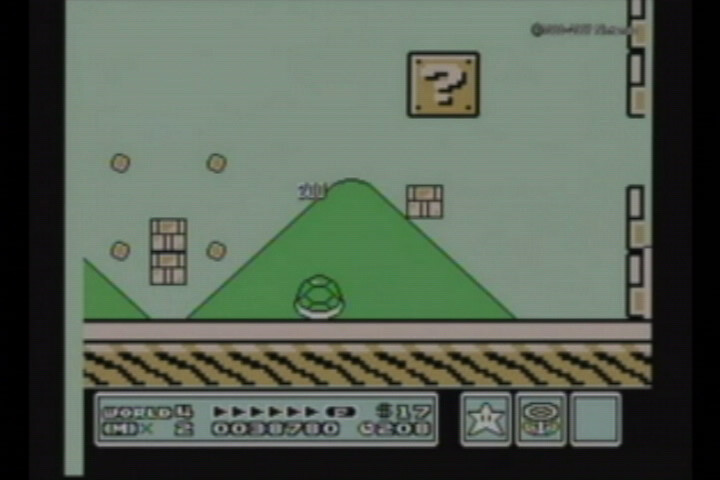This image is a detailed screenshot from the game Super Mario Brothers, likely from the third installment. The backdrop features a bluish-green sky with green triangular mountains rising from the ground, providing a classic Mario landscape. The ground itself is beige with a darker brown base, resembling soil.

On the left side of the screen, there are two small bricks stacked vertically. Above them, in the air, float several other bricks including a distinctive yellow question mark block. Near the center of the image is a green Koopa shell with the number "200" displayed in white above it, indicating that it has recently been stomped.

Additionally, near the right side of the screen, there are two tall walls with a gap between them for Mario to navigate. At the bottom of the image, it reads "World 4-2," along with a score of 38,780 points. Also displayed are three inventory boxes; one contains a star, another houses a fire flower, and the third is currently empty. The image also shows a time countdown at 2:08 and mentions $17, possibly as part of the game's coin or score system, though this detail is less clear. There are directional arrows pointing to the right, guiding the player's next move.